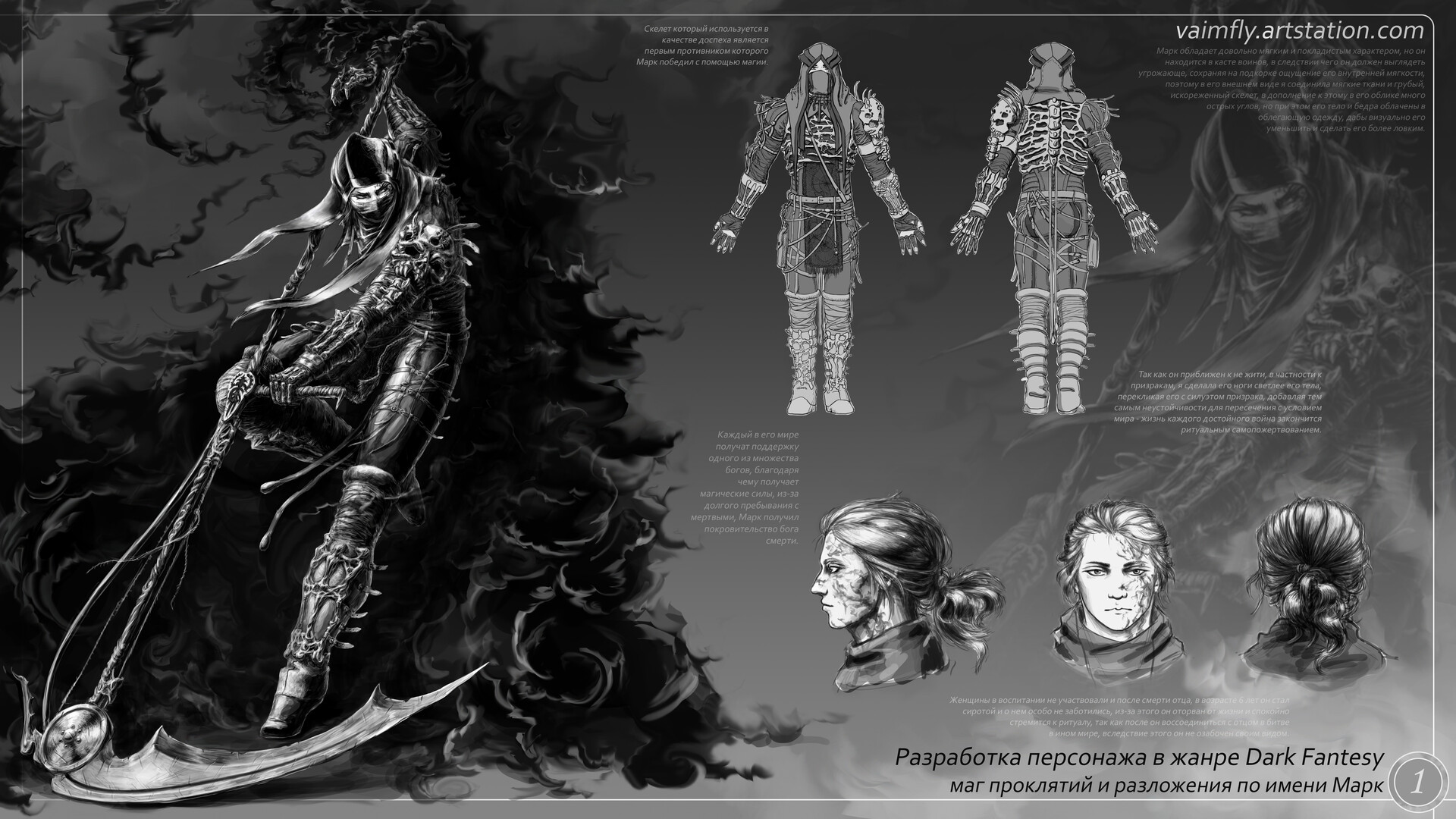The image appears to be a highly detailed character sheet, presumably for a fantasy or sci-fi-themed project like a video game or graphic novel. Rendered in black and white, the left-hand side of the artwork, which takes up about a third of the composition, features a dynamic, gothic warrior figure. This character is clad in a full leather suit adorned with numerous straps and belts, resembling a blend of fantasy and futuristic design. The warrior, likely inspired by grim reaper archetypes, wields an enormous scythe, the blade of which rests on the ground. Behind this figure, a menacing dark cloud or black flames add to the ominous atmosphere.

On the right side of the image, there are multiple detailed sketches of a female head, showcasing left profile, full frontal, and rear views. Alongside these, two futuristic, fantasy-styled robots with spiked armor are depicted. The upper right corner of the image features the website "vamefly.artstation.com", suggesting the artist's portfolio. The bottom of the page includes some text in Russian, providing additional context or information about the characters or project. Overall, the composition is rich with intricate details and conveys a strong, dark fantasy aesthetic.